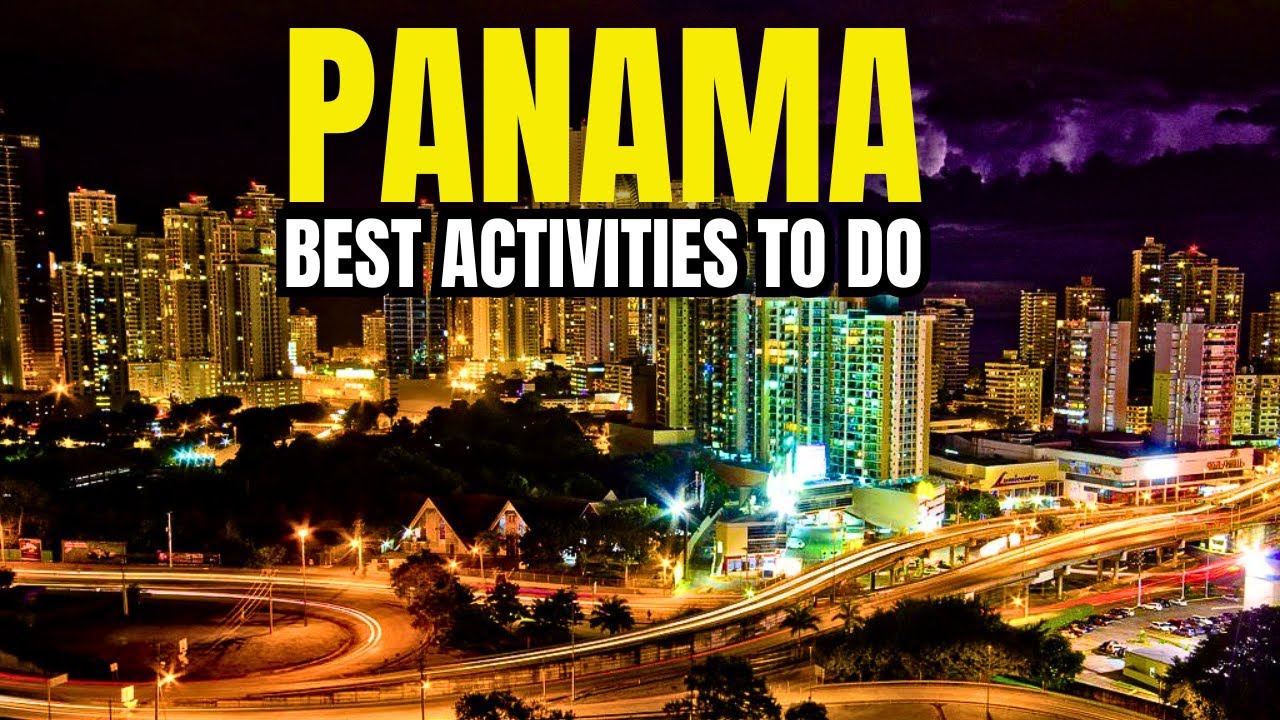A vibrant, nighttime cityscape evokes the essence of a postcard, showcasing the allure of urban nightlife. Brilliant city lights cast a kaleidoscope of colors across a bustling metropolis. In the forefront, towering buildings are adorned with vibrant lights; some emit dazzling green and red glares, while others glow with a pristine white brilliance. On the left, the sky is an inky black, transitioning to striking purple clouds on the right.

Illuminated highways crisscross through the cityscape, their lights forming dynamic trails of red, orange, and bright yellow-orange, reminiscent of the fast-paced lifestyle. These blurred lights whisk past, suggesting speed and vibrant city life, with reds and oranges near parking lots adding a fiery contrast. Flanking these arteries of light, patches of dark, leafy trees provide a natural counterpoint, with dense clusters visible in the corners and the middle of the scene.

Above this nocturnal tableau, bold yellow capital letters spell out "PANAMA," commanding attention at the top of the image. Beneath, in smaller white uppercase letters, an invitation reads: "BEST ACTIVITIES TO DO." This composition is a captivating snapshot of Panama's nightlife, blending the urban hustle with natural beauty, and serves as an alluring advertisement for nocturnal adventures in the city.